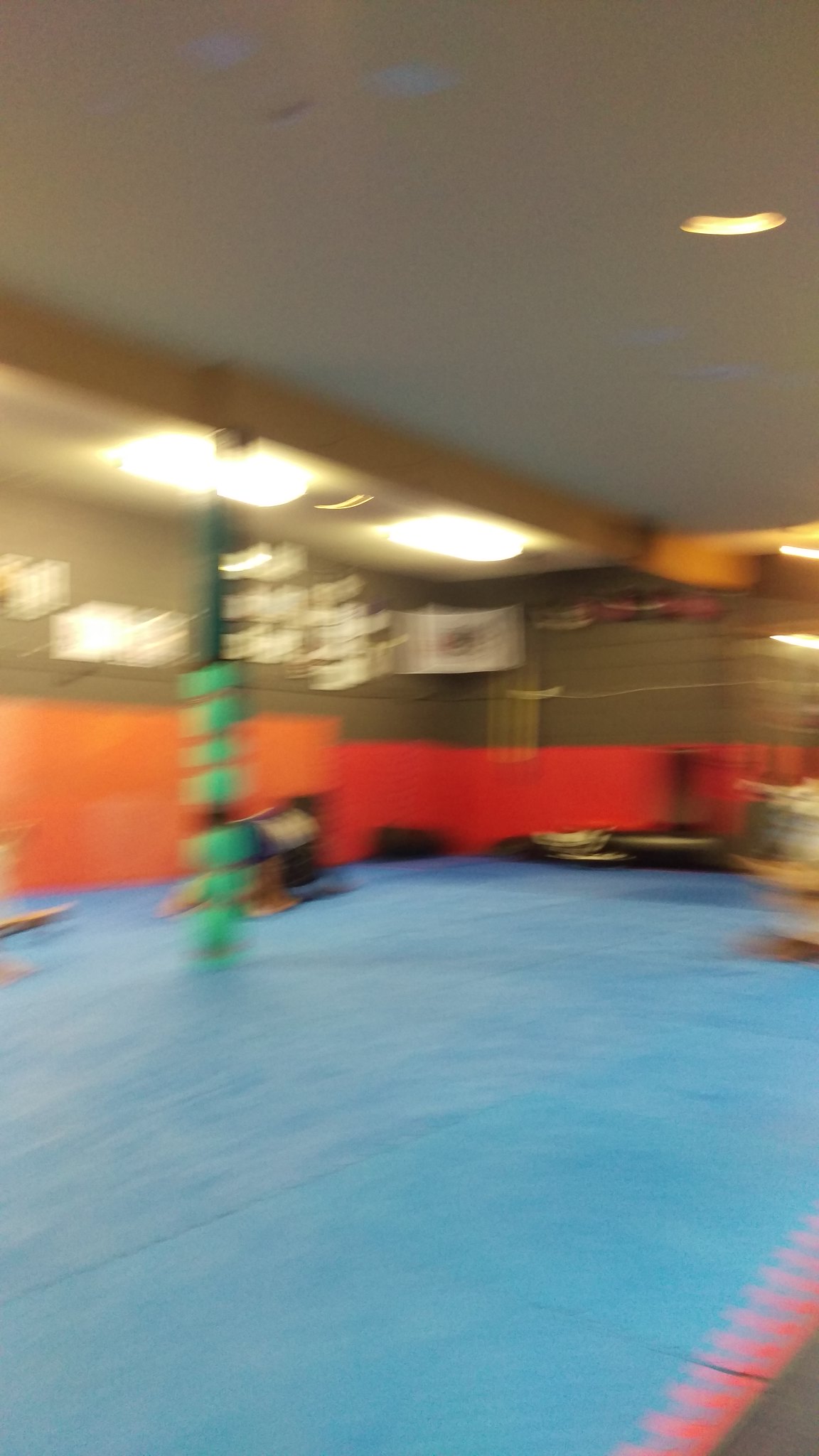In this blurry image, we can observe a gray ceiling with one prominent yellow light and two pale blue dots that could be additional light sources. There is also a section of the ceiling equipped with two rectangular fluorescent lights. Below the ceiling, a brown wall marked by some indistinguishable white elements can be seen, suggesting a large enclosed space, potentially a children's play area. 

The carpet on the floor is a light to medium blue hue. To the upper left of the carpet, there stands a pole adorned with several green objects, possibly toys or decorative items, and there may be a child partially obscured behind it. The scene includes an orange panel followed by a red panel, with the rest of the panels not clearly visible, implying that the space might be compartmentalized or partially walled off. In the lower right area of the image, it appears that the area is open, further supporting the idea that this could be a recreational or play space for children.